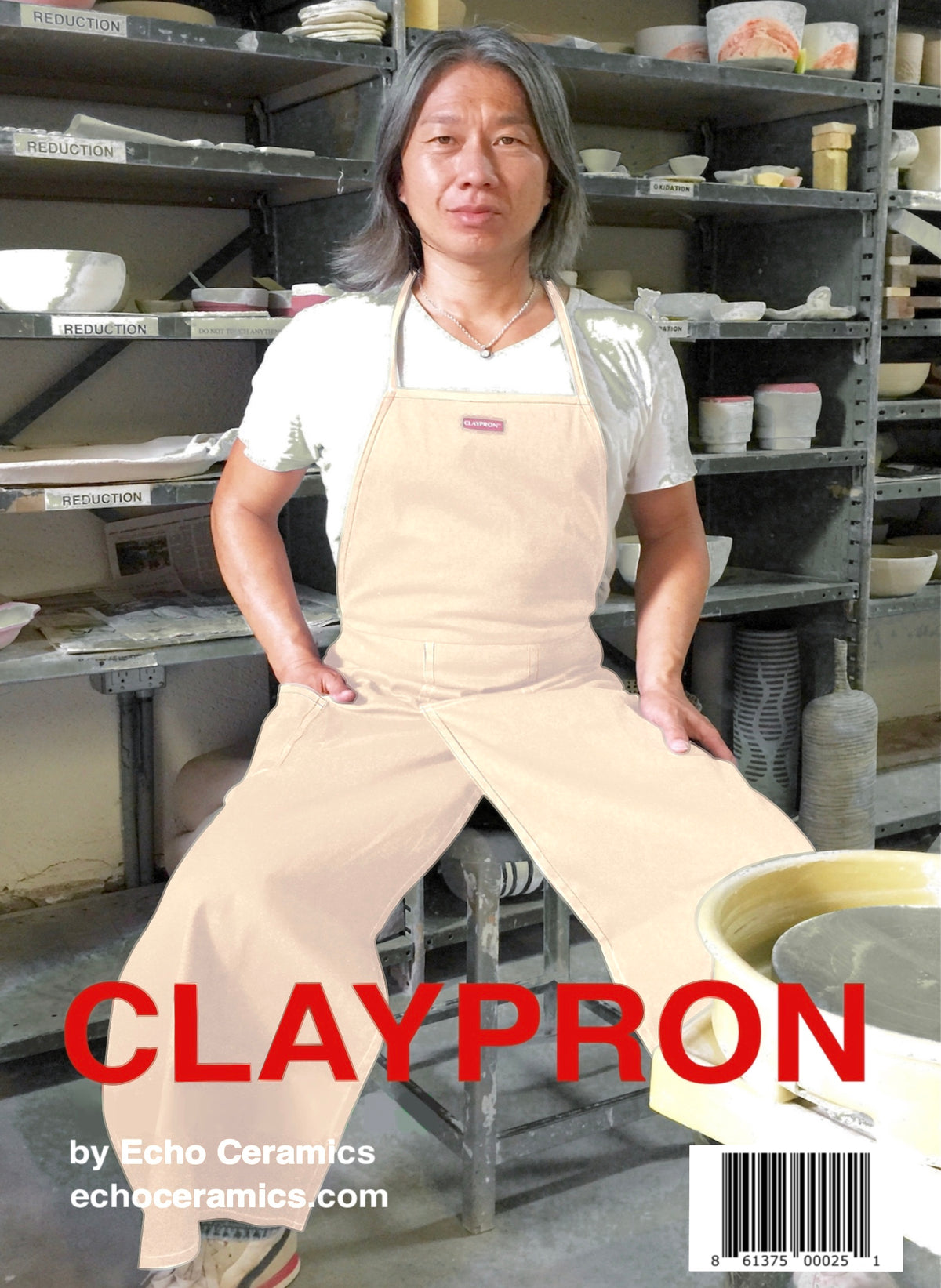The front cover of the magazine, "Claypron" (C-L-A-Y-P-R-O-N), prominently features its name in bold red lettering. Below the title, on the left side, is the website "BuyEcoCeramics.com," while a barcode, numbered 61370025, appears on the bottom right corner. The central image showcases an Asian artist—often reported as either a man or woman—posing confidently in front of a set of interconnected metal shelves loaded with an assortment of ceramic art pieces, including plates, jars, cups, and bowls. The four deep shelves have tags, with the left ones labeled "reduction" and the middle shelves possibly marked with "oxidation" or "liquidation." The artist, with shoulder-length silver hair, sports a white v-neck t-shirt, sneakers, and a beige apron that splits into two leg protectors, each with pockets. Adding to the serene workspace ambiance, the artist sits on a metal stool, gazing calmly at the camera with their right hand in the apron pocket and their left hand resting on their hip.